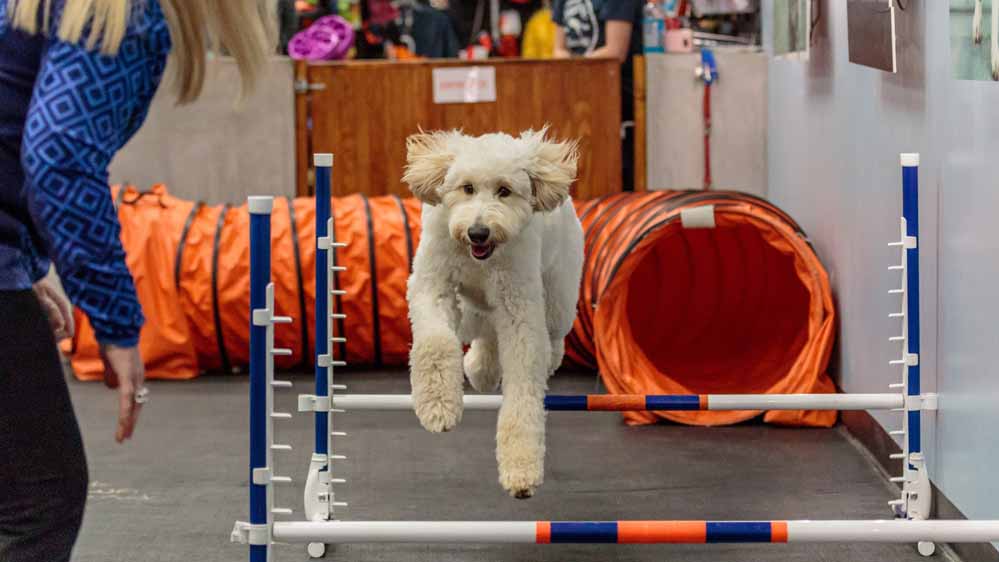The photograph captures an energetic scene of a fluffy white dog, likely a poodle mix or a labradoodle, participating in an obstacle course. The dog is in mid-jump over a set of blue and white hurdles with orange and blue stripes, its mouth open and ears flapping while its chubby paws are poised above the bars. In the background, a large orange tunnel stretches out, indicating part of the dog's training regimen. To the left side of the image, a woman with long blonde hair, dressed in a dark blue and geometric-patterned blouse and black slacks, stands encouragingly. Her attention is firmly on the dog, suggesting a deep involvement in guiding its training or performance.